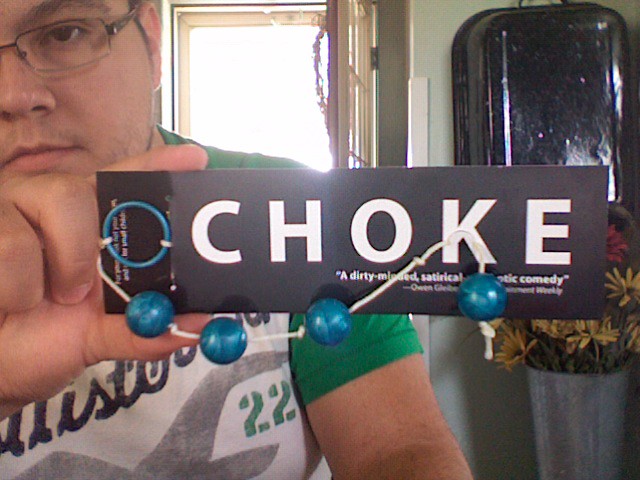In this image, a young, slightly heavyset man is photographed indoors, perhaps using a cell phone or webcam, as the picture appears grainy. He is holding up a rectangular black sign that prominently displays the word "CHOKE" in white letters. Below this, in smaller font, the sign reads "a dirty-minded satirical comedy," though part of the text may be cut off. Attached to the sign is a white string with four blue plastic beads. The man’s right hand is visible, holding the left side of the sign, and he is dressed in a white Hollister t-shirt with green sleeves and the number "22" printed on it. Only the left side of his face is clearly visible, showing his left eye, part of his glasses, nose, and lips. In the background, there is a white wall and an open door with natural daylight streaming through, revealing that the photo was taken during daytime. Additionally, a vase with fake flowers can be seen behind him.